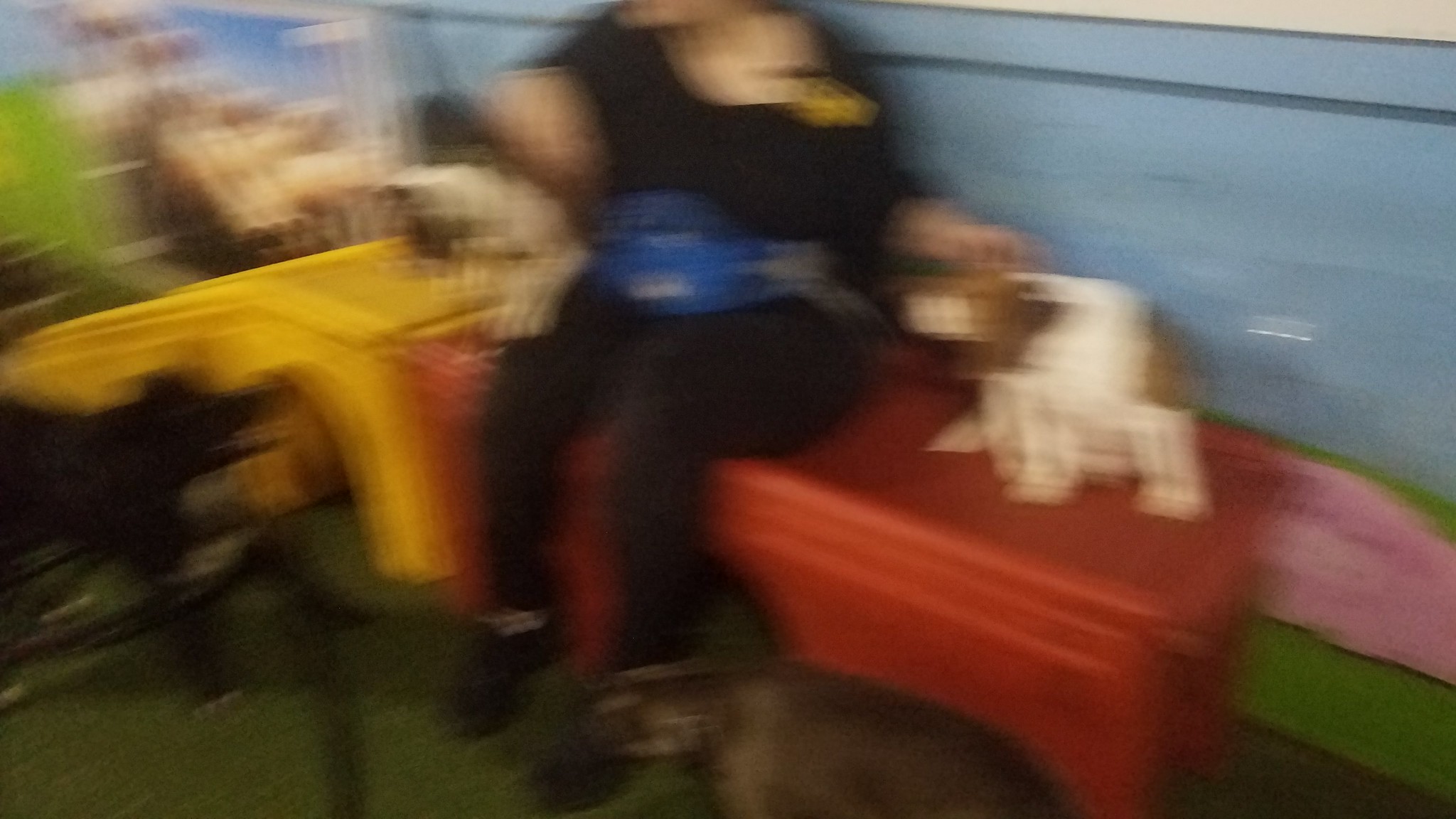In the image, a woman dressed in a black t-shirt and black leggings is seen in a semi-seated position on a small red bench, which is just large enough for two people. She is accompanied by an elderly beagle beside her. The scene is lively, with several other dogs surrounding her from all directions—front, back, and sides. To the left of the bench, a yellow slide or ramp designed for dogs leads up to the bench, adding a playful element to the setting. The atmosphere suggests a vibrant and dog-friendly environment.